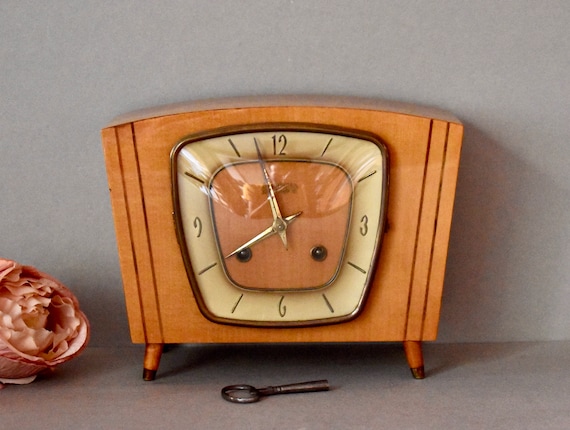The image is a color photograph featuring a vintage-style clock that resembles an old console TV set from perhaps the 1950s or early 1960s. The clock is made of light wood, with a slightly curved top and a rectangular shape. It stands on a table or counter, supported by four small peg legs. The front of the clock, resembling a TV screen, is covered with highly reflective glass and features dark gold numbers at 12, 3, 6, and 9, which indicate the time is about 11:40. The clock also has golden hands. Additionally, the clock face has stylized inscriptions on its sides and a small silver winding key at its base. Below the clock rests a small magnifying glass, and to the left, a tightly furled pink and white flower adds a touch of color. Both the table surface and the wall behind the clock are gray, providing a neutral backdrop.